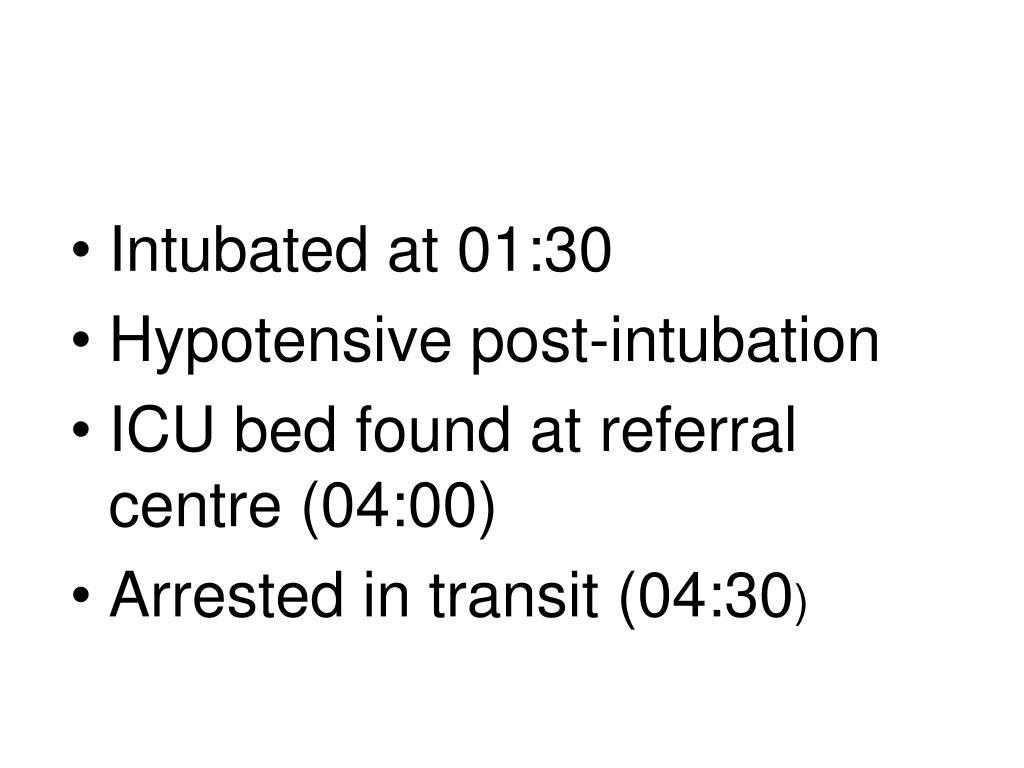This image features a clean white background with four bullet points written in black text on the left side of the page. The first bullet point says "Intubated at 01:30." The second point reads "Hypotensive post-intubation." The third point states "ICU bed found at referral center (04:00)." The final bullet point notes "Arrested in transit (04:30)." The text is black and formatted consistently throughout. There are no other objects or illustrations in the image.